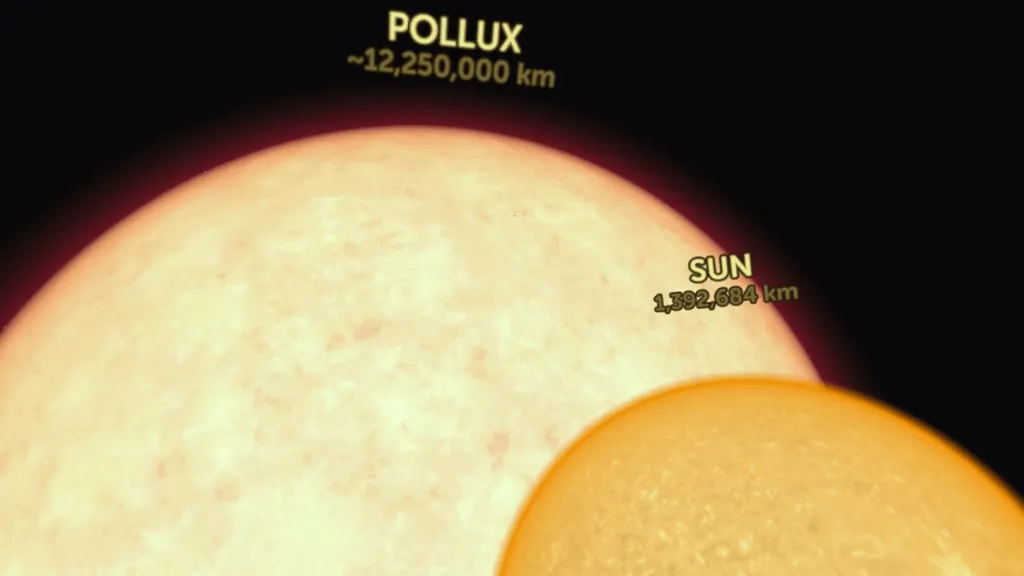This detailed image, possibly a computer-generated model or artist's rendition, depicts a size comparison between the Sun and Pollux against a jet-black space background. Positioned in the bottom right corner, the Sun, labeled with its diameter of 1,392,684 kilometers, appears as a comparatively small yellow sphere. Dominating the majority of the frame, the much larger sphere of gas identified as Pollux towers from the bottom left, taking up more than three-quarters of the visual space and labeled with its diameter of approximately 12,250,000 kilometers. The stark contrast between the sizes of the Sun and Pollux is strikingly highlighted in this vivid portrayal.